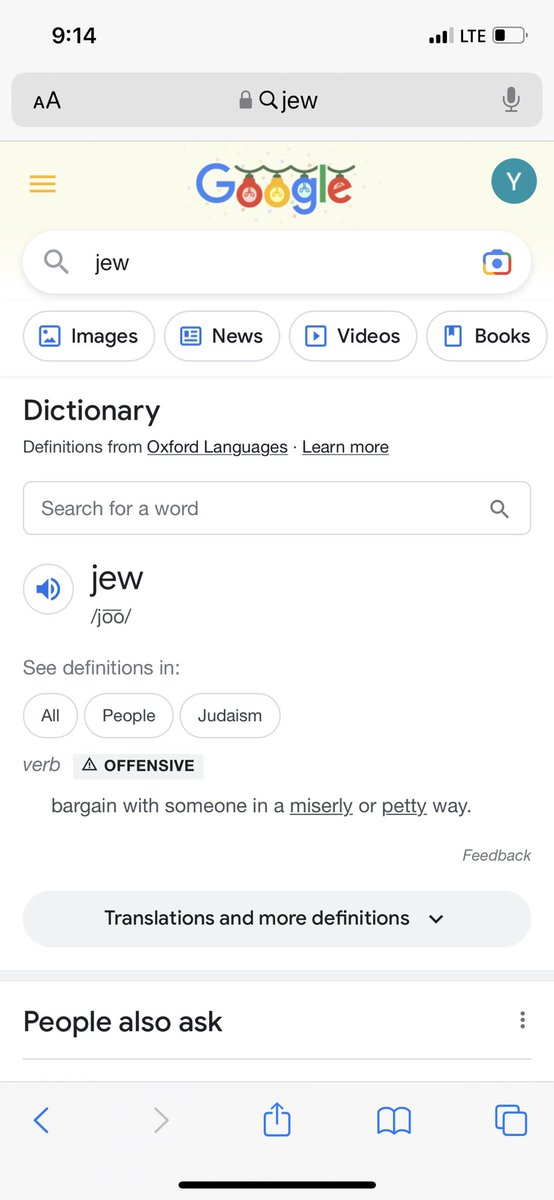This image is a screenshot taken on a smartphone, evidenced by the status bar at the top reading 9:14 for the time, with a service indicator showing three out of four bars on LTE, and a battery meter that is one-third full. The screenshot captures a Google search page where the user has searched for the word "Jew." 

Beneath the search bar, there are options for Images, News, Videos, and Books. The top result shows dictionary definitions from Oxford Languages, with options to learn more. The interface also includes a search suggestion bar, and the word "Jew" is prominently displayed below this.

The definition section provides meanings for the noun and verb forms of the word "Jew." For the verb, it states: "offensive: Bargain with someone in a miserly or petty way," highlighting its pejorative and offensive nature. This screenshot emphasizes how this usage is highly inappropriate and disparages Jewish people. 

Further down, the page includes sections for translations and more definitions, a "People also ask" segment, and navigation buttons for going back and forward, uploading, and switching to reader mode. This screenshot underscores the harmful and unacceptable nature of using "Jew" as a verb, advocating against its usage.